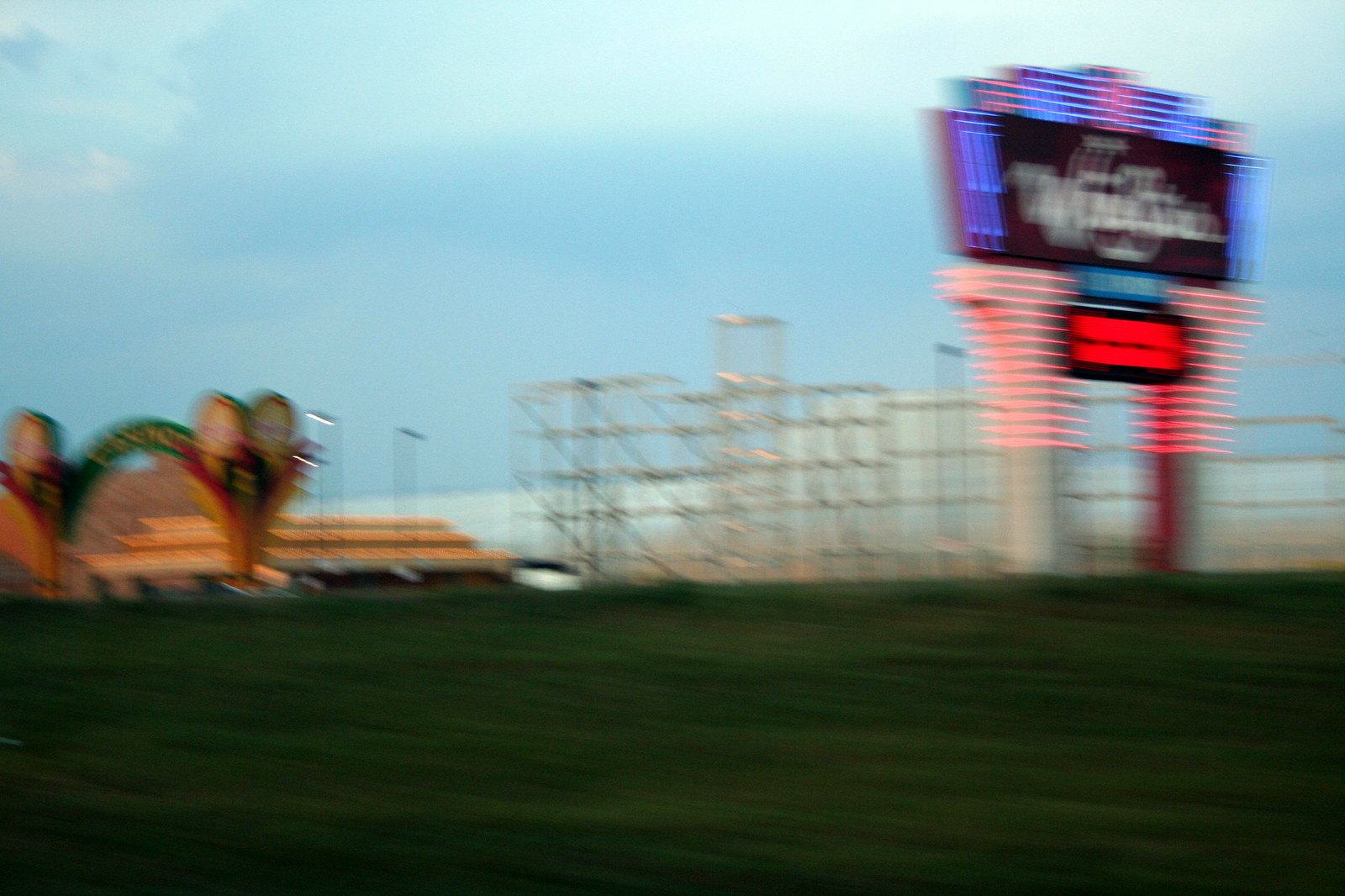This is a photograph of an outdoor scene, captured almost certainly from a moving vehicle, given its notable blurriness. The image reveals an area adorned with green grass in the foreground. Dominating the top right of the photo is an electronic marquee sign, vibrant with blue and red neon lights, most prominent at the bottom of the sign. This neon sign bridges between two columns, beneath a black sign with white text that likely indicates the name or title of the location. Adjacent to it, there appears to be scaffolding extending alongside the road.

To the left of the scaffolding stands a building outfitted with multiple neon or chaser lights accentuating its roof, which has three distinct levels. These lights, like those on the marquee, are a striking red. Fronting this structure is a large green sign featuring a yellow word arching across it. Despite the building and its surroundings being indistinct due to the image's blurriness, the numerous vibrant lights suggest it could be a casino or significant tourist attraction, reminiscent of establishments found in areas like Las Vegas or large entertainment hubs. The sky overhead is a moody, cloud-laden dusk, setting a somewhat somber yet illuminated atmosphere to the scene.